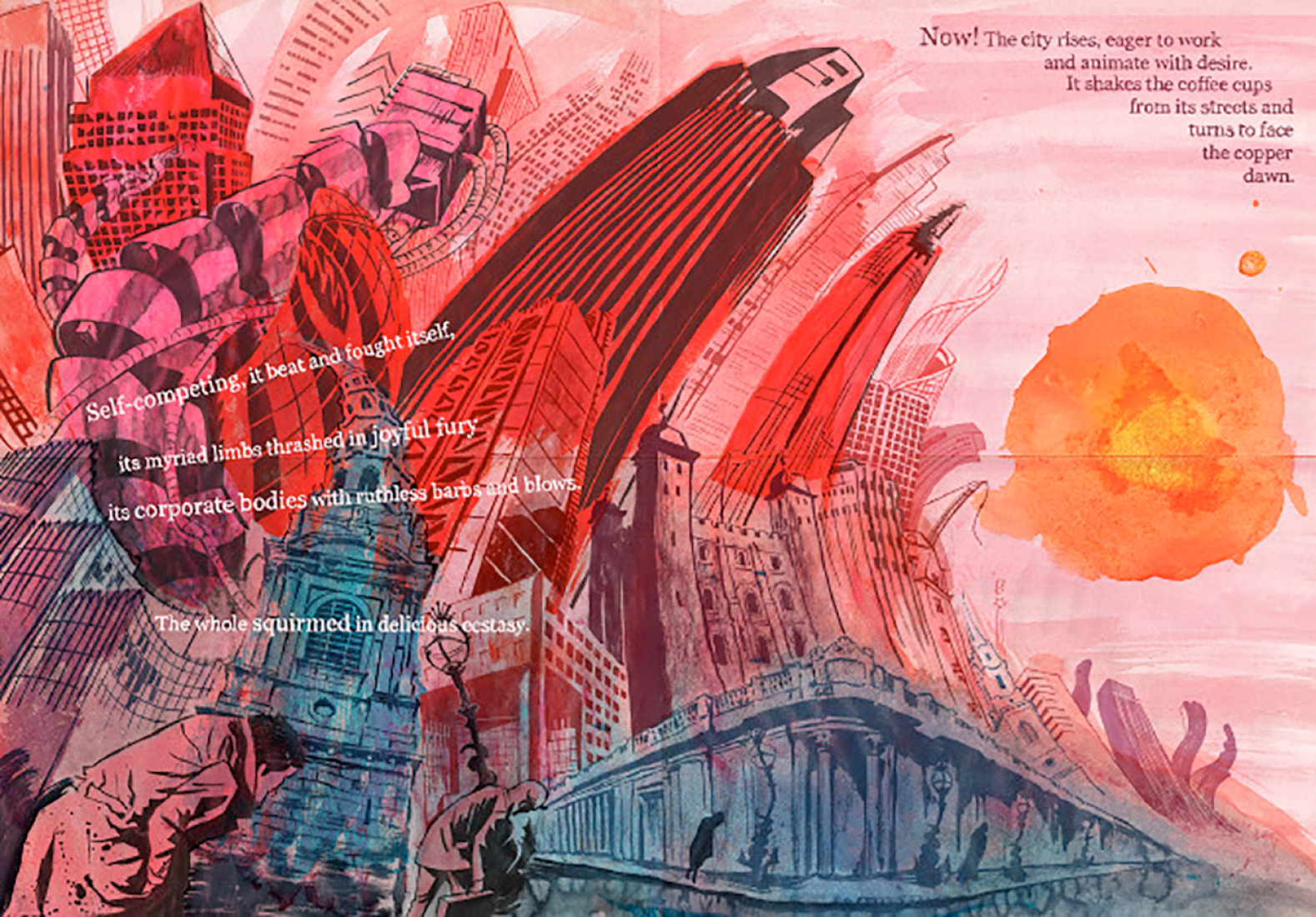This image is a vibrantly chaotic illustration, reminiscent of a comic book or graphic novel, where intense watercolor strokes of red, orange, and pink dominate the scene, punctuated by occasional splashes of blue and black. The background portrays a distressed cityscape, with tall skyscrapers curving and bending precariously in the red hues, except for one steadfast blue building standing on a city corner. In the bottom left, there is a man hunched over, donning a trench coat, seemingly ducking for cover.

On the left side of the image, inscribed text details a vivid poem: "Self-competing, it beat and fought itself. Its myriad limbs thrashing in joyful fury. Its corporate bodies with ruthless barbs and blows. The whole squirmed in delicious ecstasy." Above, the text continues, "Now the city rises eager to work and animate with desire. It shakes the coffee cups from its streets and turns to face the copper dawn." The top right portion of the illustration features what appears to be the sun, framed by skyscrapers arching towards it in eager anticipation.